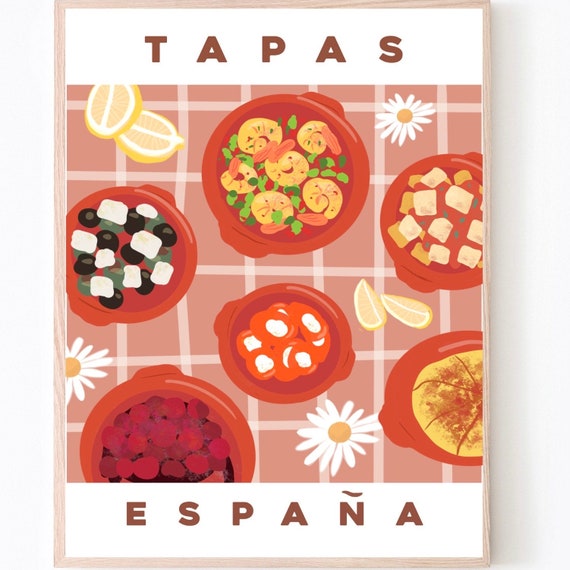The animated poster features the word "TAPAS" at the top in all caps, brown sans serif text on a white background. The main illustration showcases a pink and white checkered surface adorned with a series of six red bowls containing various Spanish tapas. The top bowl holds pieces of shrimp accompanied by a green herb. Other bowls display assorted foods including black olives with mozzarella chunks, tomato pieces with white centers, pink berries, and a yellowish square-shaped dish. Also featured is a bowl filled with red, round fruits resembling cherries. Scattered around the table are cut lemons and daisies, enhancing the inviting ambiance of the spread. The bottom of the image displays "ESPAÑA" in the same brown font as "TAPAS," signifying a focus on Spanish cuisine. The overall design is a flat vector illustration that vividly advertises the delightful variety of Spanish tapas in a cartoonish style.